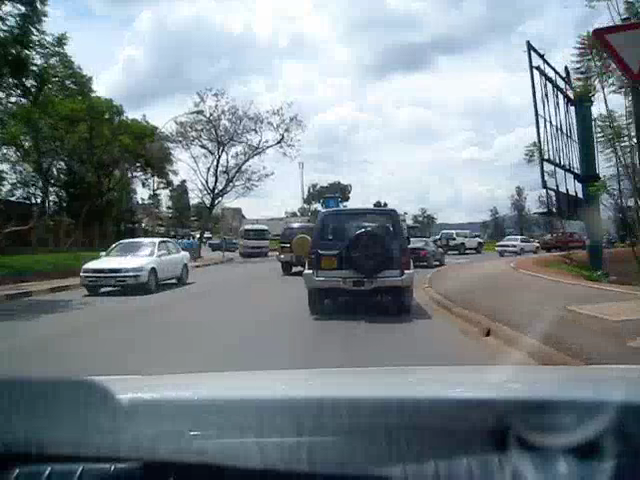This color photograph captures the view from the interior of a vehicle, looking out either the front or side window. The lower portion of the image reveals the vehicle's grey metallic interior. The primary focus of the photograph is the road ahead, where a dark black van or truck is directly in front of the vehicle, with a covered spare wheel mounted on its rear. The road curves to the right and appears to intersect with another road curving to the left, suggesting a junction. 

Further along the road, a white car approaches from the left side, followed by a white van. The left side of the road is lined with green grass and trees, while the right side features a pavement and a large black gate. A street sign with a white background and red edge is partially visible on the right. The sky above is predominantly overcast, with patches of blue peeking through the cloud cover.